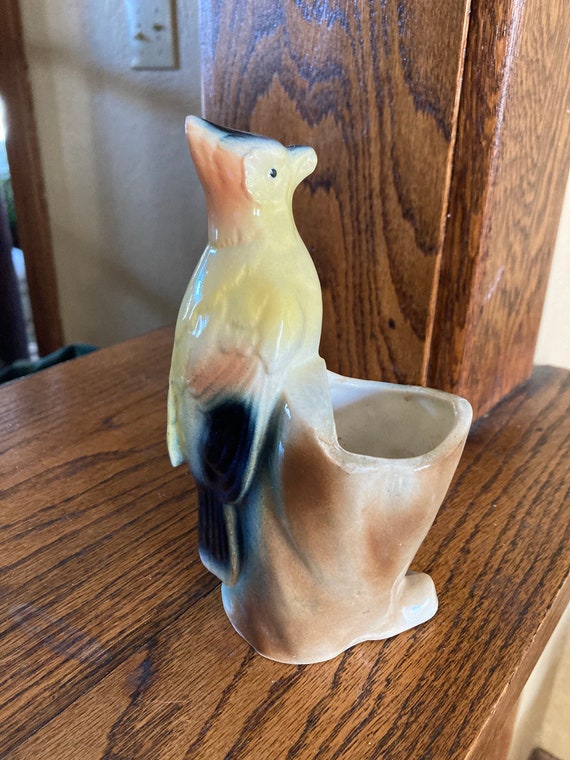The photograph is a detailed, color portrait of a ceramic bird sculpture standing on a wooden countertop. The bird, which has vibrant yellow feathers transitioning to orange on its head and black on its tail, appears to be perched on what resembles a cut tree trunk or an exaggerated shoe. This structure, possibly broken or intentionally designed, doubles as a functional container with a cup-like shape and a white interior, suitable for holding flowers, pencils, or other items. The scene is set against a background that includes a wooden post and a light switch in the upper left quadrant, enhancing the household atmosphere. The entire arrangement sits at a comfortable arm's length from an average adult standing beside it.